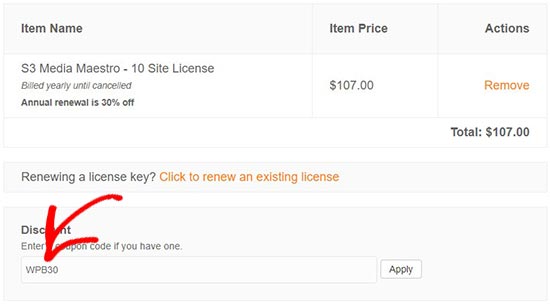This image is a screenshot from a website or app displaying a billing or checkout interface. At the top, there is a table with a header row containing three columns: "Item Name," "Item Price," and "Actions," all written in black bold print on a light gray background. 

The second row is white with black text, except for the "Actions" column which has red text. The "Item Name" column reads "S3 Media Maestro, 10-site license, billed yearly until canceled," followed by "Annual renewal is 30% off" in bold. The "Item Price" column displays "$107," and the "Actions" column includes a "Remove" option in red text.

The third row spans the entire width of the table and displays "Total: $107" in bold lettering.

Below this table, there's a light gray bar that invites users to renew a license with the prompt, "Renew a license key, click to renew an existing license." Adjacent to it, another gray row offers a discount section with the text "Discount, enter coupon code if you have one," followed by a field pre-filled with "WPB30" and an "Apply" button.